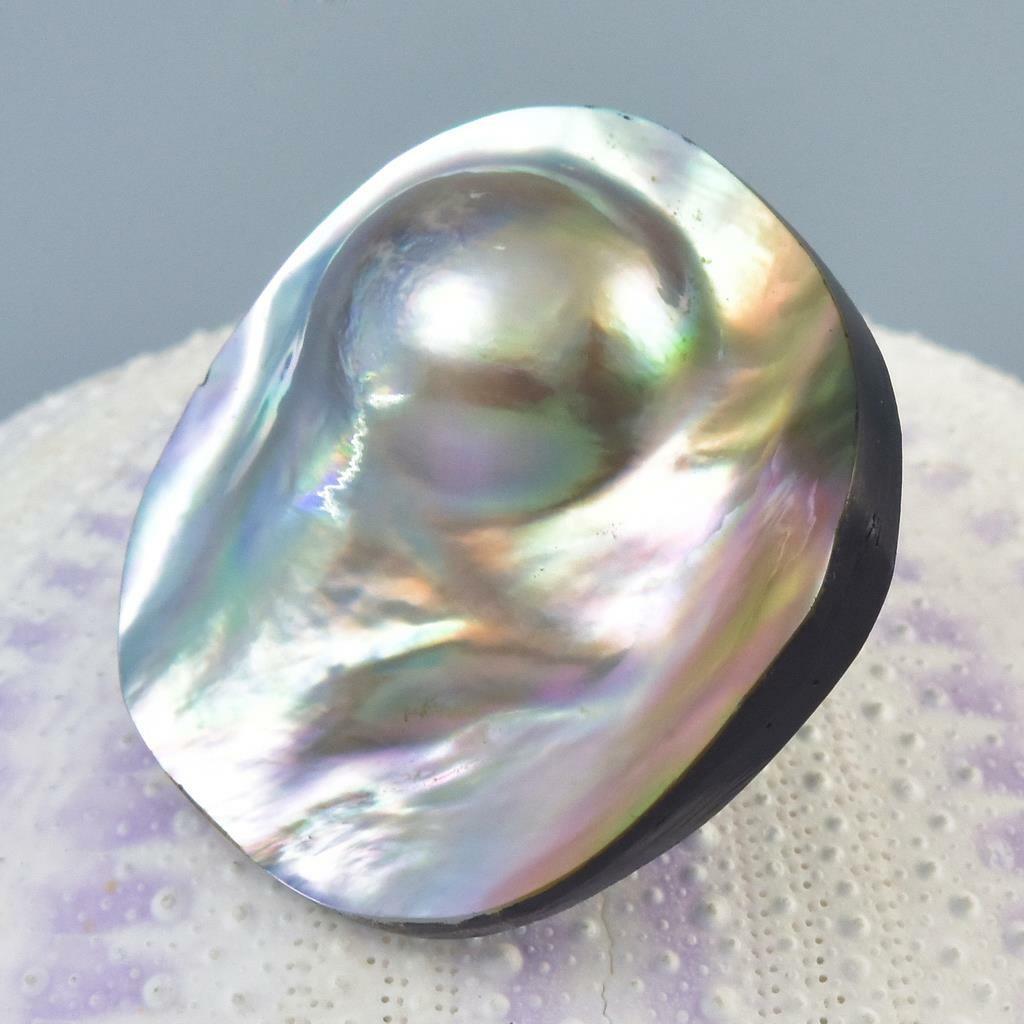This photograph captures a detailed close-up of what appears to be a blister pearl embedded in a clam shell. The pearl has a distinct metallic sheen, reflecting hues of silver, purple, lavender, blue, and light green, which gives it a vibrant, almost iridescent appearance. The pearl itself is characterized by a round bulge that emerges from the upper center of the shiny, oval-shaped, metallic surface, reminiscent of abstract art or jewelry. This central bulge is the recognizable, lustrous part customarily associated with pearls. The shell beneath the pearl is bumpy, primarily white with pink spots, and possibly a clam or abalone shell, suggesting a textured, natural setting. The backdrop of the image is a blue wall, enhancing the shell and pearl's vivid coloration. The pearl and shell rest on a purple and white sphere with circular indentations, contributing to the artistic and intricate aesthetic of the scene. There are no additional objects visible in the photo, keeping the focus entirely on the pearl and its shell.